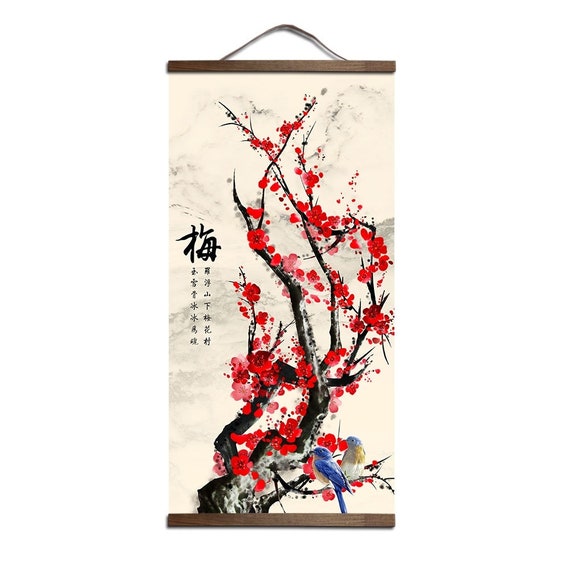A vertical, rectangular artistic piece, reminiscent of a Japanese scroll from the Sengoku era, hangs from a visible wire on a wall. The piece, framed by wooden borders at the top and bottom, is mounted on an off-white, beige background. Dominating the scroll are vivid multi-color elements including reds, pinks, blues, blacks, and browns. Prominently, on the left side, large Japanese characters are alongside smaller inscriptions, perhaps offering inspirational messages. In the lower right, two birds - one light blue and the other a darker blue - perched on a branch adorned with red, white, and pink blossoms, add a lively touch to the otherwise serene composition.